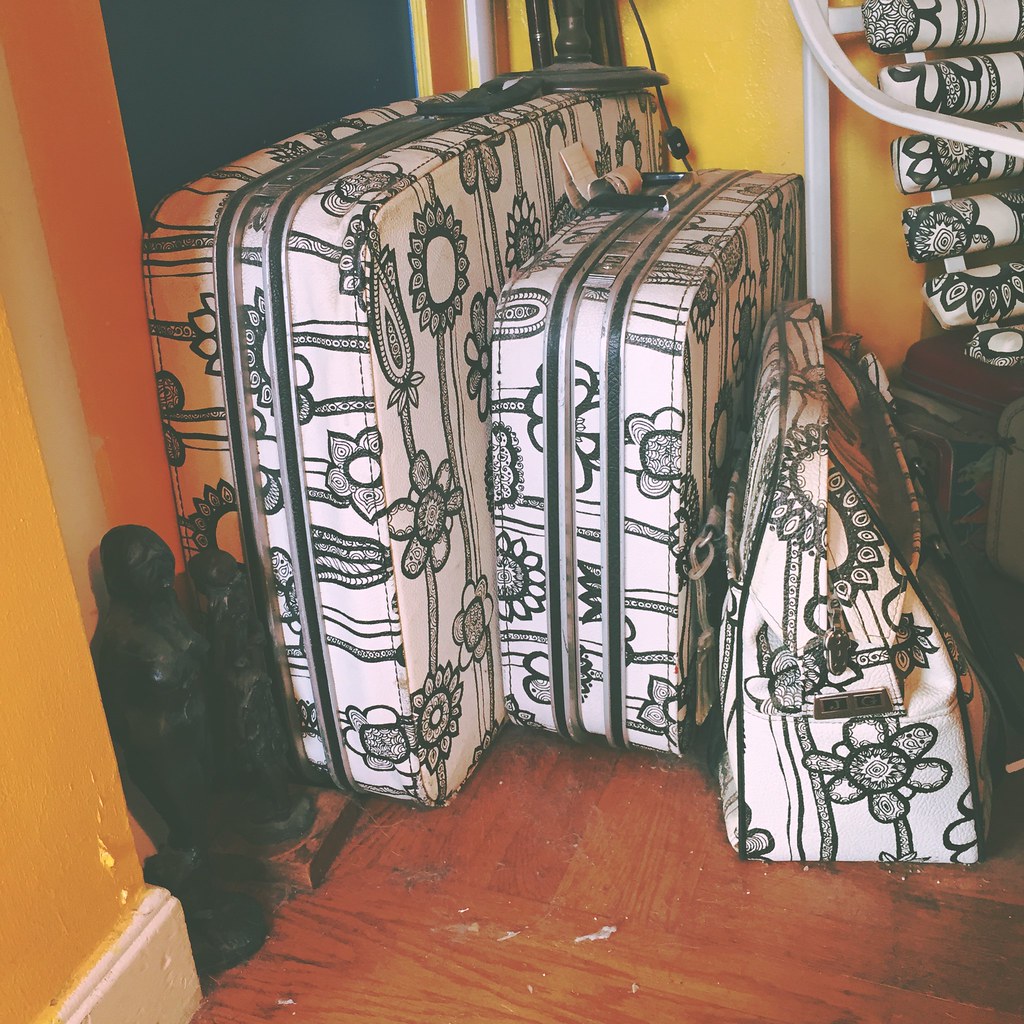The image depicts a set of three matching pieces of luggage positioned on the wooden floor against a vibrantly painted wall. All three bags feature a striking black and white floral pattern with detailed design elements repeated on each item. The set consists of a large suitcase on the left, a medium-sized briefcase in the center, and a smaller accessory that resembles a purse on the right. Accompanying these bags are two miniature black statues that resemble tribal figures, situated to the left of the luggage. The floor appears dusty and dirty, emphasizing a rustic setting. The background wall is painted in a mix of yellow, red, and blue hues, adding a colorful backdrop. Additionally, to the right of the luggage, there are hints of the same black and white floral pattern on what seems to be rolls of fabric or possibly a chair decorated with the same design, integrating the luggage set into the overall decor.